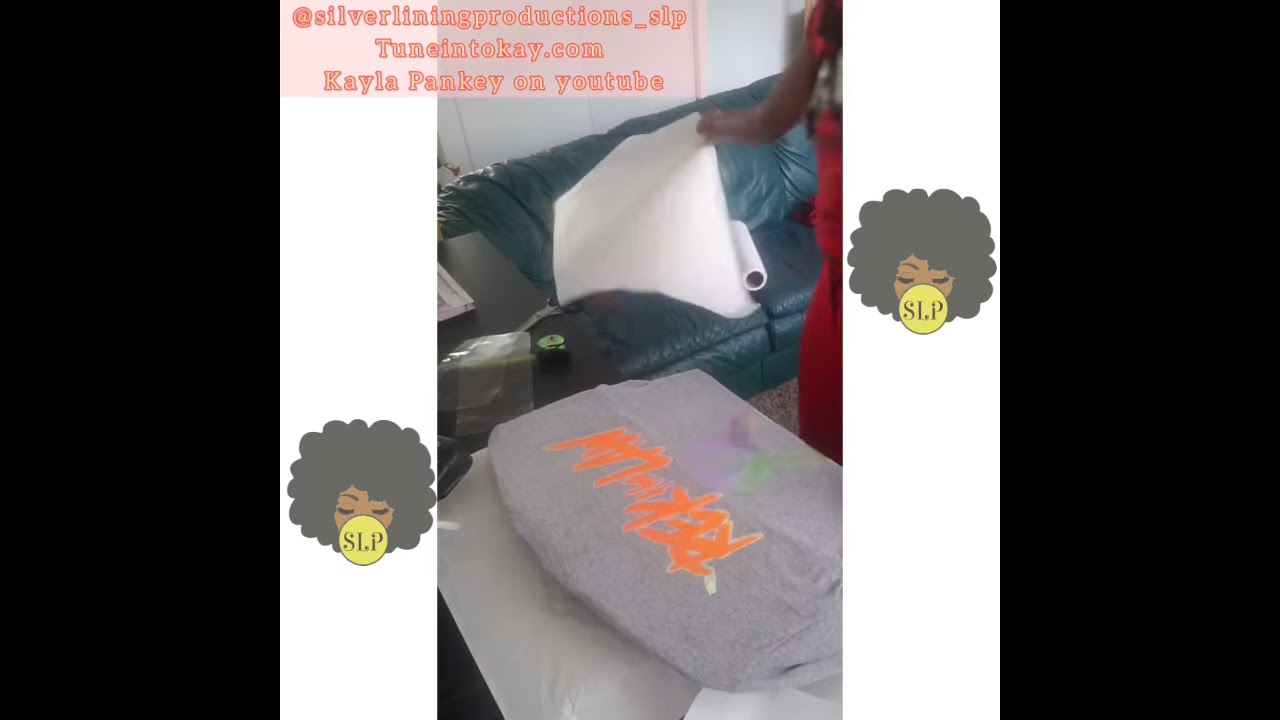The indoor photo captures a dynamic scene with an African-American woman in motion, situated to the right-hand side, partially cut off. Her dark skin and attire—a red outfit with a cartoon-styled logo—complement the setting. She is unrolling a large sheet of paper towel while leaning against a teal, turquoise-blue leather couch. This couch serves as the background, along with a white wall.

In the foreground, a light grey sweatshirt with orange graffiti-style text is noticeable, though upside down and angled. Scattered around are items indicative of crafting or cleaning: scissors, tape, a bag, and other clothing articles.

Promotional text overlays the top of the image, reading "at silverliningproductions_SLP, tuneintokay.com, Kayla Pankey on YouTube," and vertical white bars on either side feature illustrations of a black woman with a large afro and the letters "SLP" on a yellow circle near her mouth. The combination of these elements suggests the image’s use for social media promotion, specifically to highlight Kayla Pankey’s online presence and her YouTube channel.